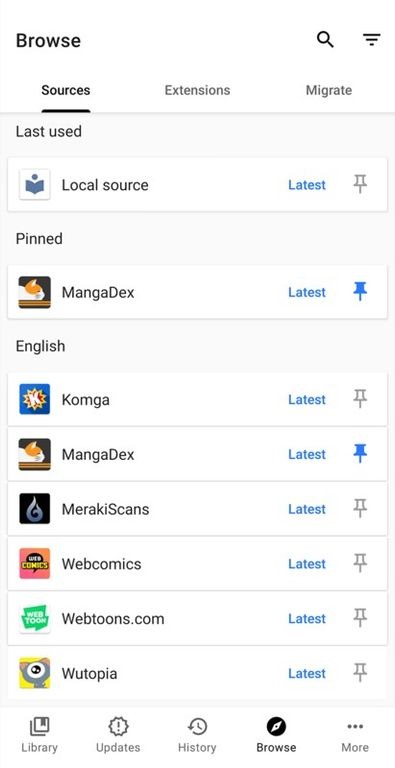The image appears to be a user interface of a digital reading platform, adorned with various options and icons:

1. Top left corner displays the word "Browse."
2. Upper right corner features a magnifying glass icon and a WiFi symbol.
3. Below these, the word "Sources" is prominent and underlined in black.

Below the underlined "Sources," there is a navigation bar with options:
- "Extensions"
- "Migrate"

Beneath this bar:
- A gray rectangle labeled "Last Used."
- Below this, a white rectangle titled "Local Source" with the text "Latest" in red and blue. It also includes a thumbtack icon labeled "Pinned."

Further down, there are various listings:
1. **Magnadeex (Cat head icon)**
   - Label: "Latest" in blue
   - Blue thumbtack icon
   - Language: "English"
   
2. **Core Conga**
   - Pattern with a "K"
   - Label: "Latest"
   - Gray outline thumbtack icon
   
3. **Magnadeex (Cat head icon)**
   - Label: "Latest" in blue
   - Blue thumbtack icon

4. **Merit Key Scans**
   - Black square with a silver design
   - Label: "Latest" in blue
   - Gray thumbtack icon
   
5. **Web Comics**
   - Peach colored background with yellow and black text
   - Label: "Latest"
   - Gray thumbtack icon
   
6. **Webtoons.com**
   - Green speech bubble icon
   - Label: "Latest" in blue
   - Gray thumbtack icon
   
7. **Wutopia**
   - Yellow box, resembling cat's ears and an eye
   - Label: "Latest"
   - Gray thumbtack icon

At the bottom of the section, the following items appear:
- "Library" with stacked pages icon.
- "Updates" with a gear shift or starburst design featuring an exclamation point.
- "History" with a circular icon containing an arrow and clock hands.
- "Browse" in a black circle with a white design inside.
- "More" with three dots.

This image effectively showcases the interface's structure, emphasizing key features and organizational elements for a seamless browsing and reading experience.